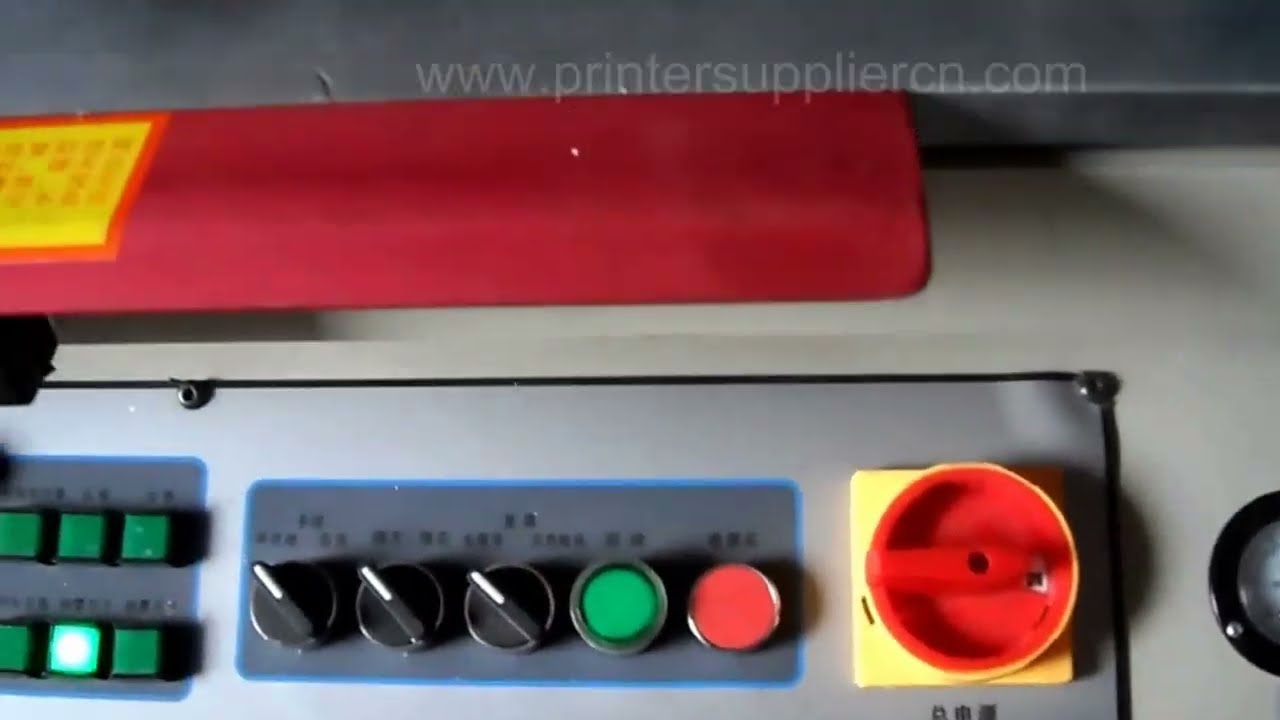This image showcases a detailed control panel of a commercial piece of equipment. At the top, in white letters, is the website www.printersuppliercn.com. Below this, a red bar spans the width of the image. On the left side of the panel, there are six square green buttons arranged in two rows. Moving right, three black knobs with white tips are aligned horizontally in the center of the panel, which appear to be tactile and adjustable. To the immediate right of these knobs, there is a smaller round green button and a similarly sized red button. Further right is a larger recessed red dial with a yellow square base around it, designed to be twisted. The panel itself is gray and features a silver plate with visible screws and rivets securing it in place. The image suggests that the equipment is likely used in an industrial or commercial setting.